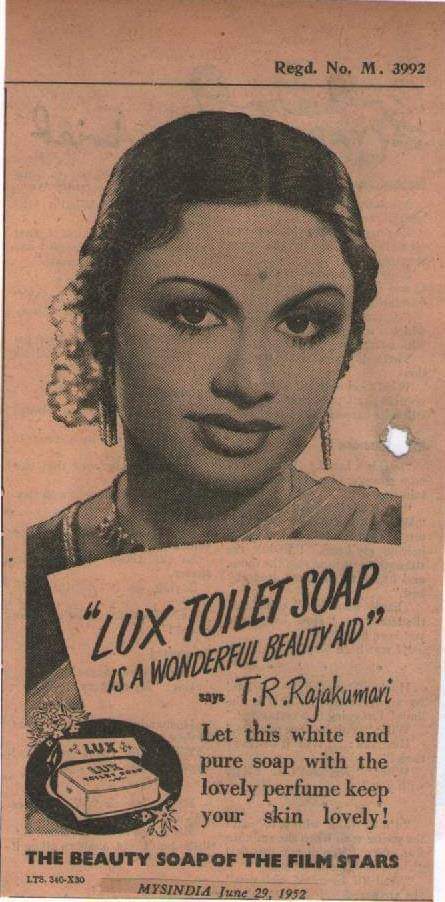This image captures a vintage newspaper advertisement from June 29, 1952, featuring a prominently displayed photograph of a beautiful Indian woman, adorned in traditional attire including a gown, intricate necklaces, and earrings. The aged newspaper, with its yellowed and orange-tinted paper, showcases a vivid blend of black and white imagery against a brownish-reddish backdrop. Central to the ad is an endorsement by T.R. Rajakumari, stating, "Lux Toilet Soap is a wonderful beauty aid." Accompanying this declaration is a description praising the soap's pure and perfumed qualities, encouraging users to "keep your skin lovely." To the left of the woman's image is an illustration of a Lux soap bar, emphasizing its association as "The Beauty Soap of the Film Stars."